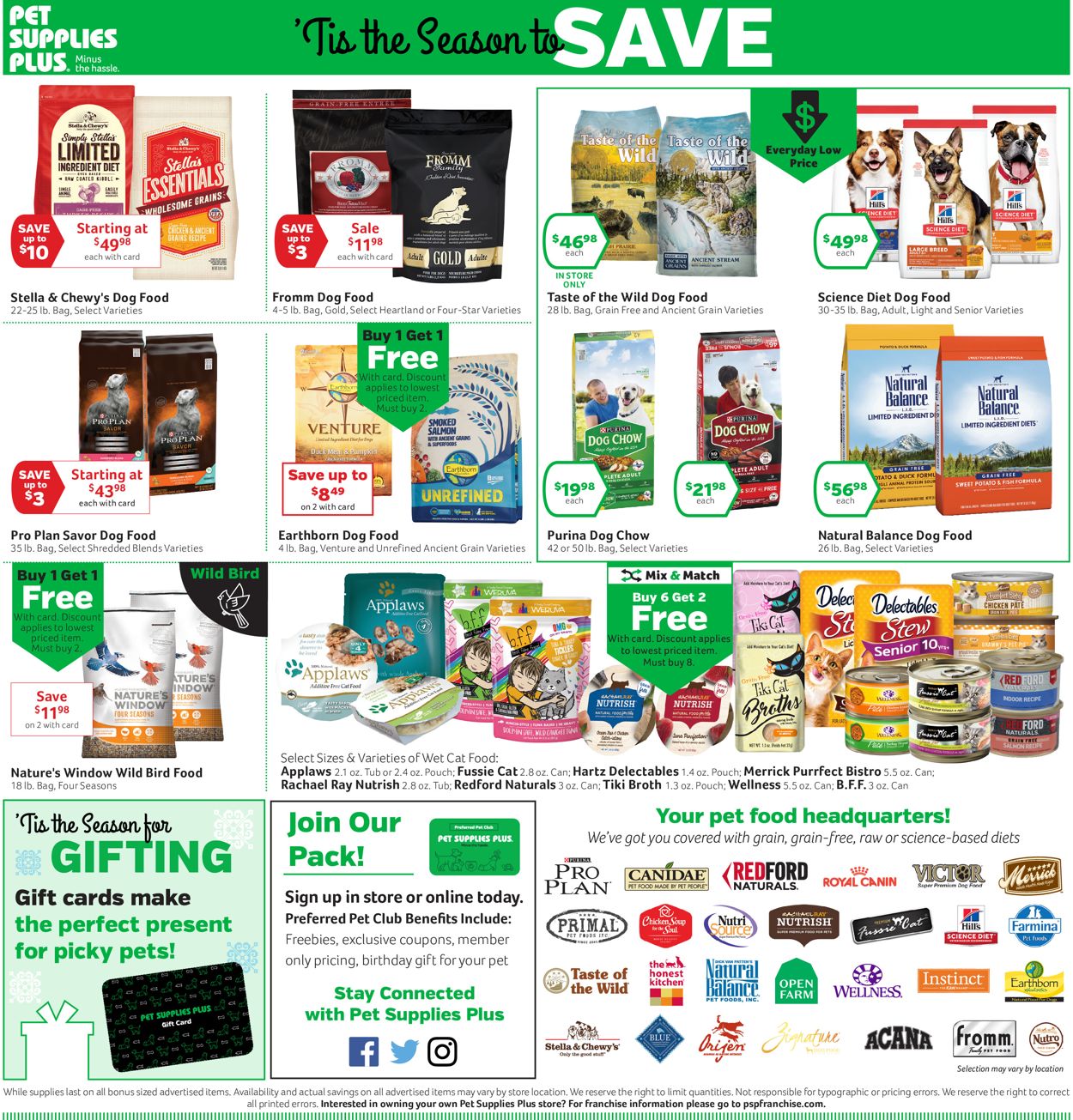The image showcases a collection of store coupons prominently branded with "Pet Supplies Plus" in white text at the top left corner, accompanied by the slogan "Minus the Hassle" in smaller lettering to its right. Dominating the top middle section is a festive banner reading "Tis the Season to Save," with "Tis the Season to" in black and "Save" in white.

Beneath this banner, various pet products are displayed within individual boxes. The top left box features "Stella and Chewy's Food" with images of a red bag and a light brown bag of pet food. Directly to its right, another box advertises "From Dog Food" in two black bags. 

On the top right, a larger section is divided into four smaller areas, each showcasing different dog foods: "Taste of the Wild Food" in the top left, "Science Diet Dog Food" in the top right, "Purina Dog Chow" in the bottom left, and "Natural Balance Dog Food" in the bottom right.

At the bottom left corner of the image, a highlighted box exclaims "Tis the Season for Gifting" alongside a message that "Gift cards make the perfect present for picky pets," illustrated with an image of a gift card. Just to the right of this, another box invites customers to "Join Our Pack" with the instruction to "Sign up in-store or online today."

The overall layout is designed to attract pet owners with a variety of promotional offers and gift ideas for the holiday season.